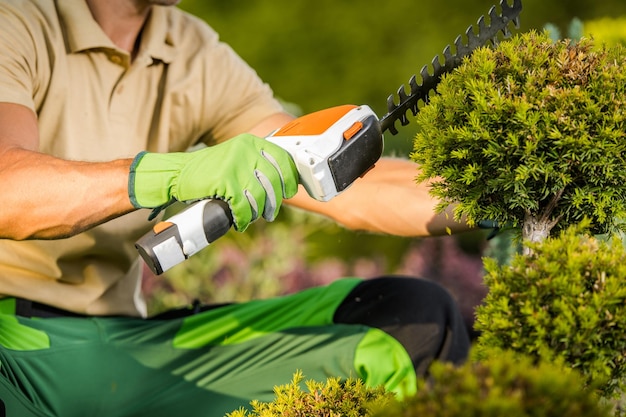In the photo, a tanned, muscular man is engaged in yard work, likely trimming a bush with vibrant green leaves. He is holding a white and orange electric device equipped with a blade, designed for precise cutting. His attire includes a light beige, short-sleeved polo shirt and dark green pants, complemented by lime green safety gloves. The man's posture suggests he is either standing or crouched while carefully maneuvering the tool. The background features a variety of blurred plants and trees, adding a lush, verdant backdrop to his gardening activity. Notably, his face is cropped out, focusing the attention on his concentrated efforts and well-defined arms, veins visible due to his tanned skin.